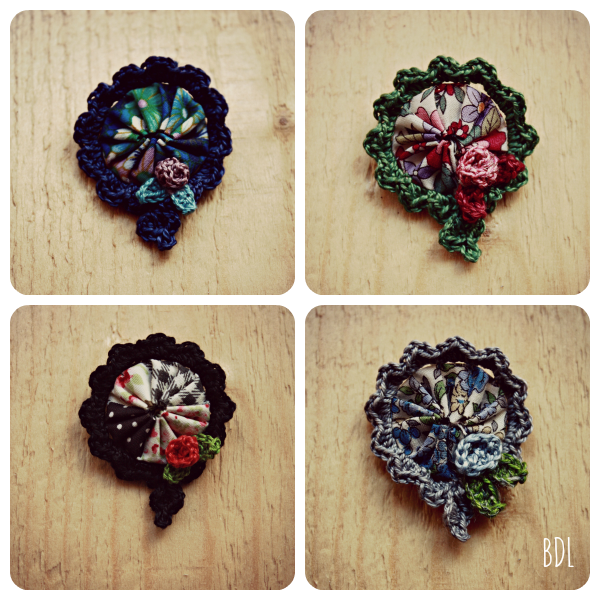The image features four quadrants, each presenting a close-up of a crafted circular brooch-like knickknack, akin to items commonly found on Etsy or similar artisan shops. Each piece, carefully arranged for display on a wooden table, is made from a combination of knitted and fabric components. The outer border of each item is a gathered, weaved fabric creating a miniature wreath effect, adorned with a crocheted flower in the lower right-hand corner.

The top left quadrant features a brooch with a blue and green knitted border, enclosing a floral fabric design in shades of blue and green. The top right quadrant displays a green-knitted border with a red and white floral pattern, accented by a red and pink crocheted flower. The lower left quadrant presents a black-knitted border with a fabric in black and white plaid and polka dots, accompanied by a red rose flower. Lastly, the lower right quadrant showcases a brooch with a blue and green knitted border and a floral fabric pattern in lighter shades of blue and green, featuring a white flower. The initials "BDL" are inscribed in white letters in the lower right corner of the fourth quadrant.